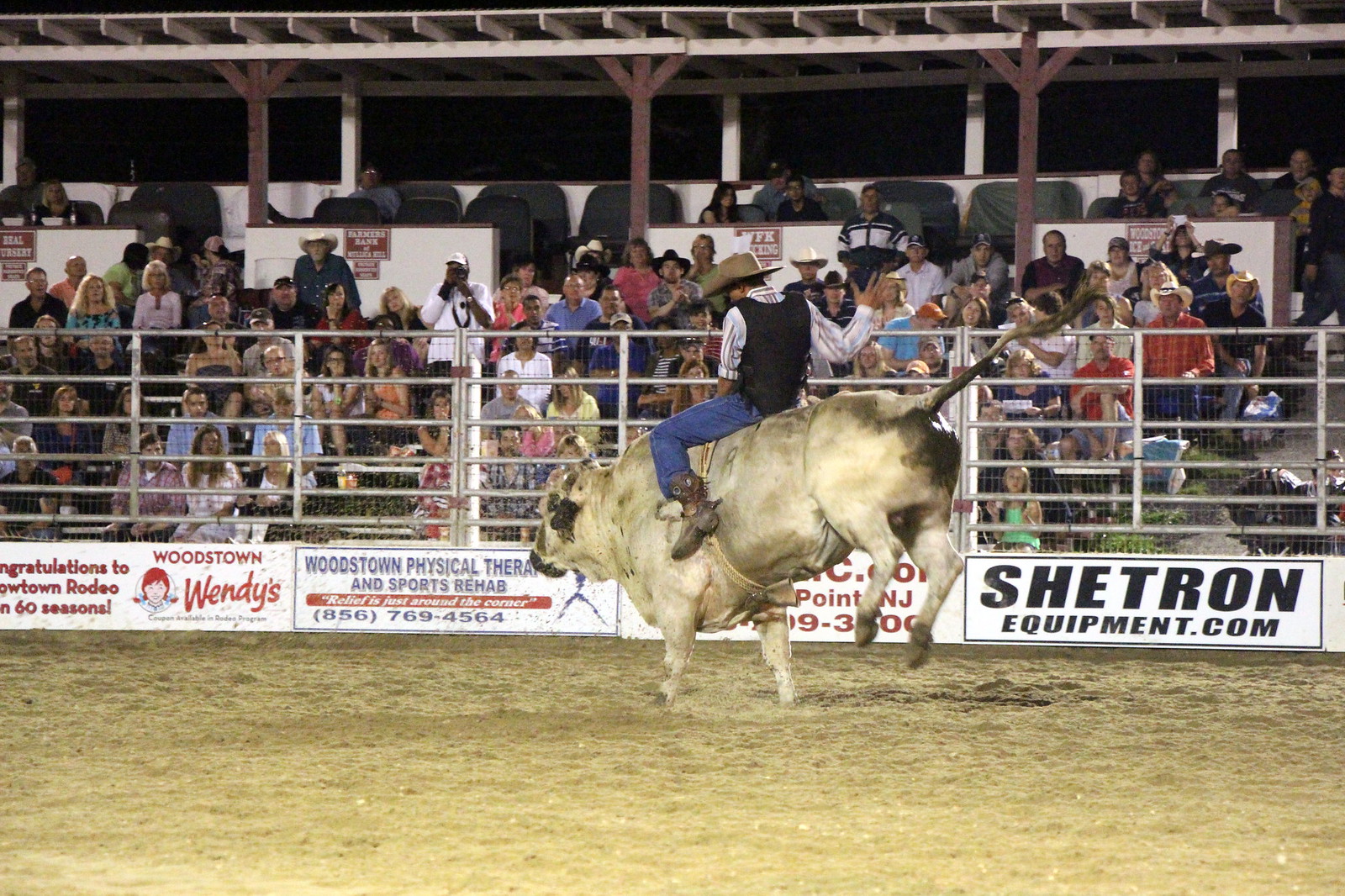The image captures a dynamic moment at a rodeo, featuring a man riding a bucking bull with a distinctive white and gray coat, black hind end, dark brown and black tail, and black accents around its ears and mouth. The cowboy, dressed in blue jeans, brown cowboy boots, a black vest, a white and dark-colored striped long-sleeve shirt, and a tan cowboy hat, is gripping a harness tightly as the bull leaps, its hind legs flailing in mid-air. The arena floor is a light tan sandy dirt, and a silver metal fence separates the action from the spectators. The audience, seated in the wooden stands under a silver roof supported by brown beams, is a colorful mix, with many wearing cowboy hats in black and white, and clothes in various hues including white, black, blue, pink, red, and green. Among the spectators, children are also visible. Advertisements line the bottom wall of the arena, displaying brands like "Woodstown Wendy’s" in red on a white background, "ShetronEquipment.com" in black, and "Woodstown Physical Therapy and Sports Rehab" along with a contact number in blue on a white background. The scene captures the excitement and vibrant atmosphere of a rodeo event.